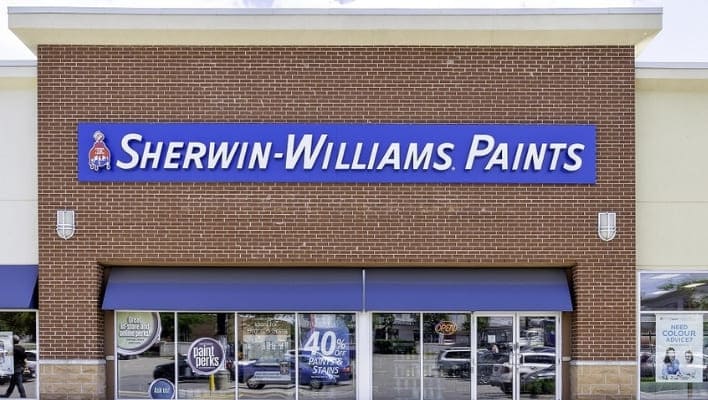The image showcases the exterior of a Sherwin-Williams paint store. The building features a flat-topped roof and a robust brick façade. Dominating the front wall is a prominent Sherwin-Williams sign, with large white letters set against a vibrant purple background. Below the sign, there's a graphic of paint spilling from a paint bucket. The lower portion of the wall is lined with multiple windows adorned with promotional signage. One of the signs advertises "Paint Perks: 40% off paints and stains," while another sign indicates that the store is open. Towards the far right of the image, there's a notice offering color advice. A person is seen walking out on the left side, likely toward the parking lot visible in the foreground. The entrance doors lie beneath a blue awning that tops the display windows. The reflections of parked cars can be seen gleaming off the windows and doors, adding a dynamic element to the scene.